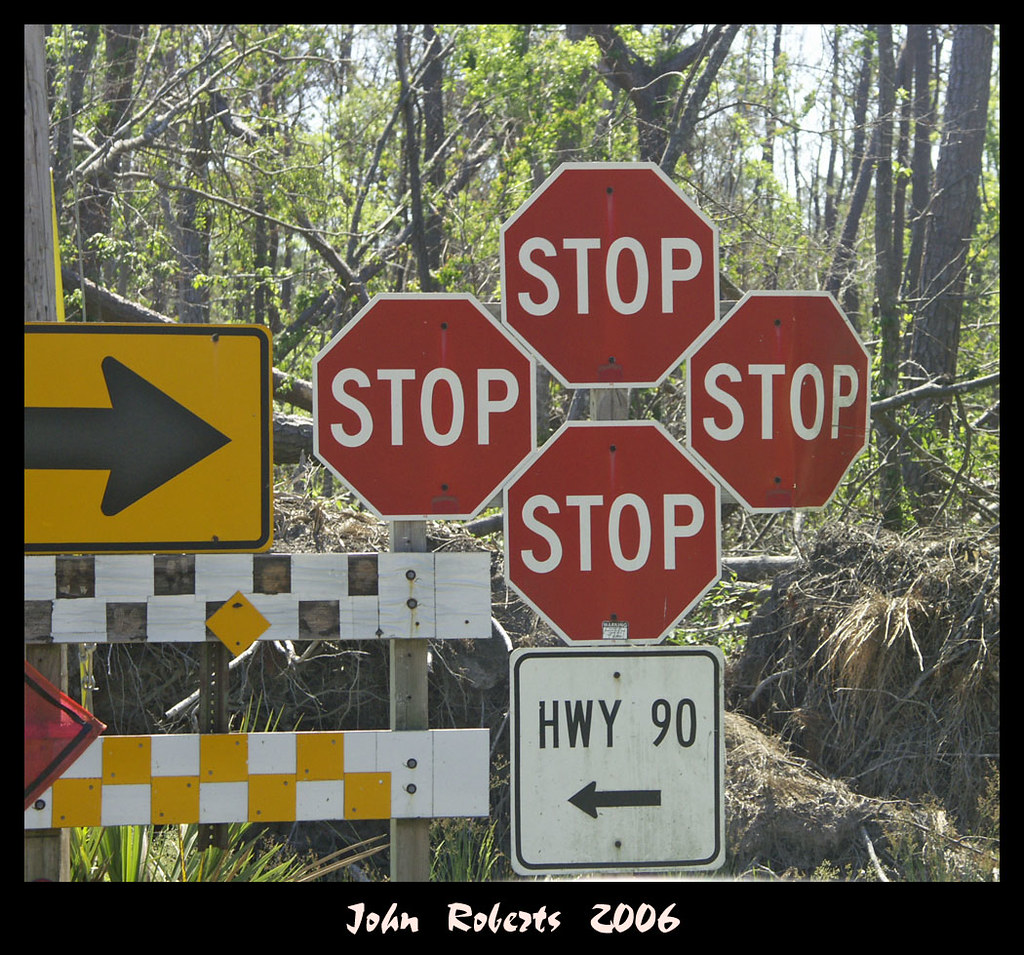This photograph, taken by John Roberts in 2006, captures an outdoor scene in a heavily wooded area with tall trees, green leaves, and abundant branches under a sunny, clear sky. Central to the image is a cluster of street signs. Dominating the composition are four stop signs, arranged in a diamond or circular pattern. Below them is a white sign edged in black, reading "HWY 90" with an arrow pointing to the left. On the left side of the frame, there's a partially visible yellow sign with a black arrow pointing to the right. Underneath this yellow arrow sign, a barrier or roadblock features two boards: the upper board displaying a black-and-white checker pattern, and the lower board a yellow-and-white checker pattern. The bottom of the photograph has a black border with the text "John Roberts, 2006" inscribed in white.